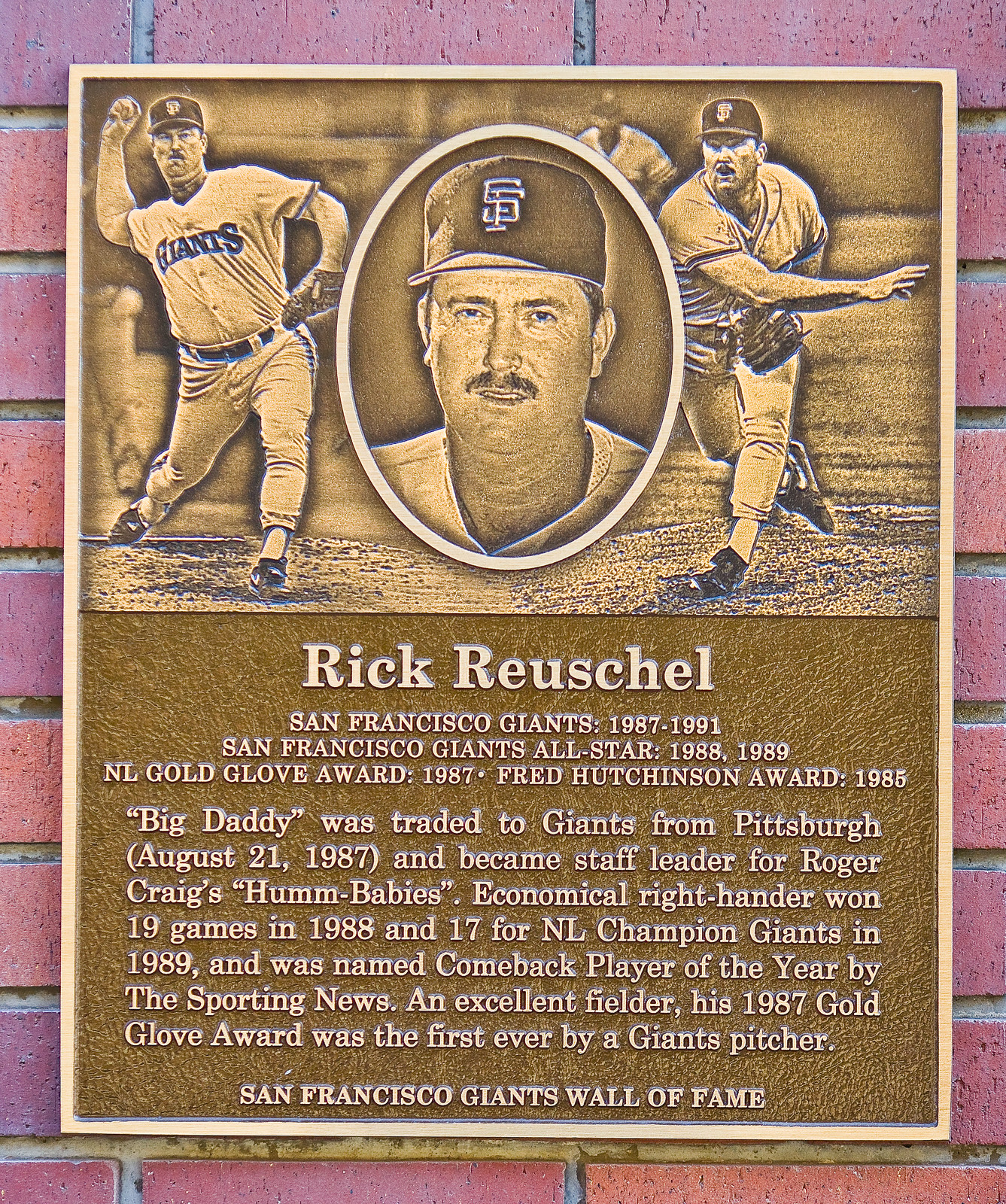This intricate bronze plaque is mounted on a pristine red brick wall with gray sealant between the bricks. At the top of the plaque is a central oval portrait of Rick Reuschel, a San Francisco Giants player, wearing a red San Francisco Giants hat and sporting a mustache. The portrait is flanked by two images depicting him throwing a baseball. The text on the plaque reads: "Rick Reuschel, San Francisco Giants 1987-1991, San Francisco Giants All-Star 1988-1989, NL Gold Glove Award 1987, Fred Hutchinson Award 1985." Below this, it elaborates: "'Big Daddy' was traded to the Giants from Pittsburgh on August 21, 1987, and became staff leader for Roger Craig's 'Hum Babies.' An economical right-hander, he won 19 games in 1988 and 17 for NL Champion Giants in 1989, and was named Comeback Player of the Year by the Sporting News. An excellent fielder, his 1987 Gold Glove Award was the first ever by a Giants pitcher." At the bottom, it affirms his place on the "San Francisco Giants Wall of Fame."